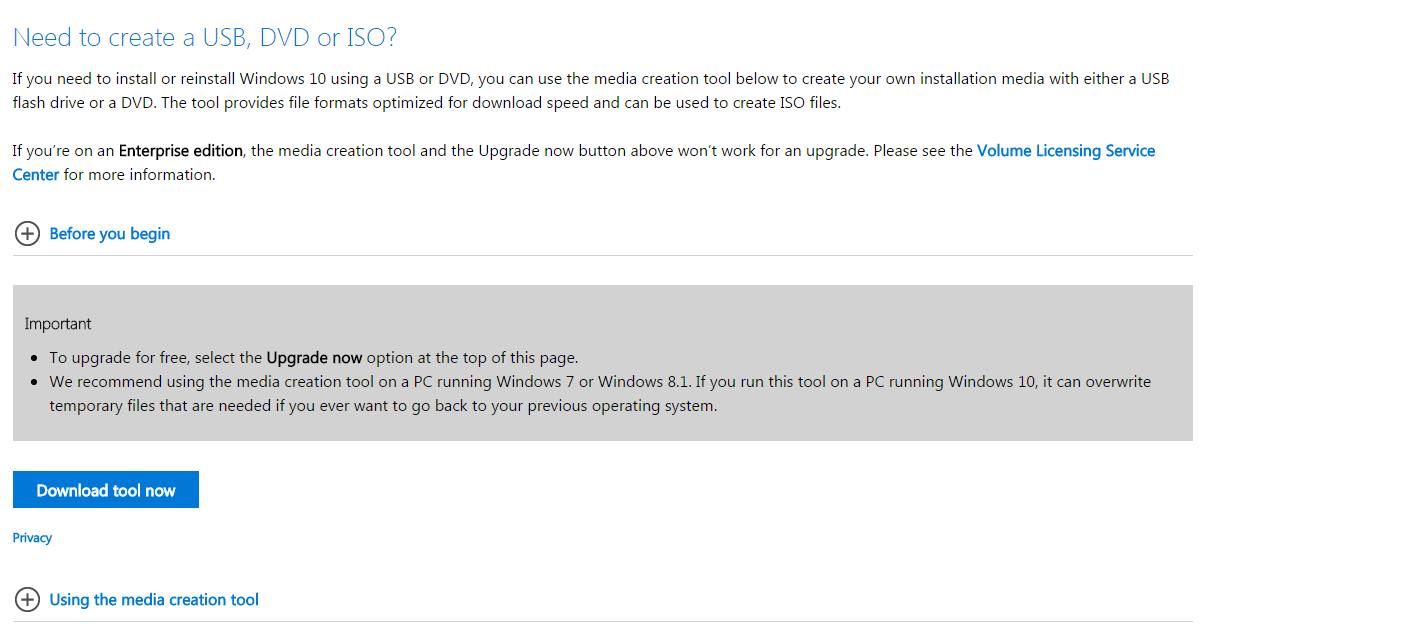**Image Caption: Detailed Instructions for Creating Windows 10 Installation Media**

The image falls under the category of websites and features detailed instructions for creating Windows 10 installation media. Predominantly, it displays a webpage with prominent blue lettering at the top that reads, "Need to create a USB, DVD, or ISO?" The instructions provided are specifically for people looking to install or reinstall Windows 10 using these mediums.

Key points highlighted include:
1. **Overview**: You can use the media creation tool below to create installation media such as a USB flash drive or DVD.
2. **Capabilities**: This tool offers formats optimized for download speed and can also be used to create ISO files.
3. **Enterprise Edition Notice**: A bolded note states that if you are using Windows 10 Enterprise Edition, neither the media creation tool nor the 'Upgrade Now' button will work for an upgrade. Instead, users are directed to the Volume Licensing Service Center for additional information.

Further down in the instructions, there are cautions and recommendations:
- **Pre-requisite Info**: Before beginning, it’s important to note that for a free upgrade, you should select the 'Upgrade Now' option found at the top of the page.
- **Recommended System**: The guide recommends using the media creation tool on a PC running Windows 7 or 8.1. Running this tool on a Windows 10 PC could overwrite temporary files necessary for reverting to your previous operating system.

At the conclusion of these instructions, the image features a prominent blue button labeled "Download Tool Now," guiding users to initiate the media creation process. The overall design aids users in creating installation media while offering necessary warnings and guidelines to ensure a smooth process.